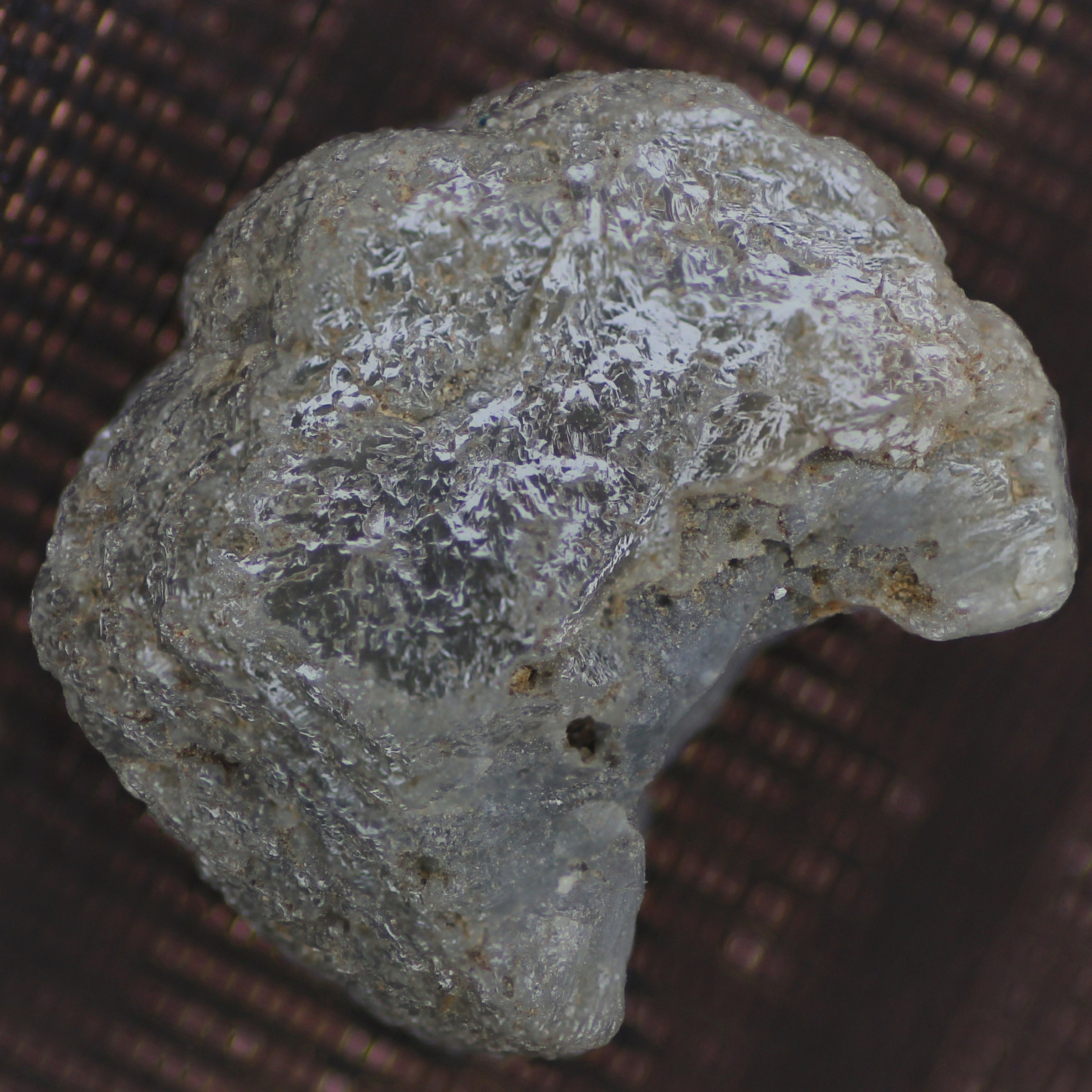The image presents a shiny, lumpy object that is predominantly silver with a metallic sheen. Its irregular, almost half-moon shape features both rough and smooth areas, adding to its enigmatic texture. The object, resembling either a piece of crumpled tinfoil or a rock with a metallic finish, appears on a background that blends various shades of brown and reddish-brown. This background, possibly a woven basket or a dark brown box, contains indistinct patterns of squares and circles, though it is somewhat blurry and unclear.

The close-up, slightly aerial perspective of the image reveals the silver object, which possesses a smoky gray cast, contributing to its ambiguous and potentially moldy appearance. This cast may hint at old, spoiled food remnants within the tinfoil-like structure. Despite the lack of textual context, the detailed view emphasizes the contrasting shiny and dull aspects of the object, while the intricate backdrop adds a layer of complexity to the overall composition.